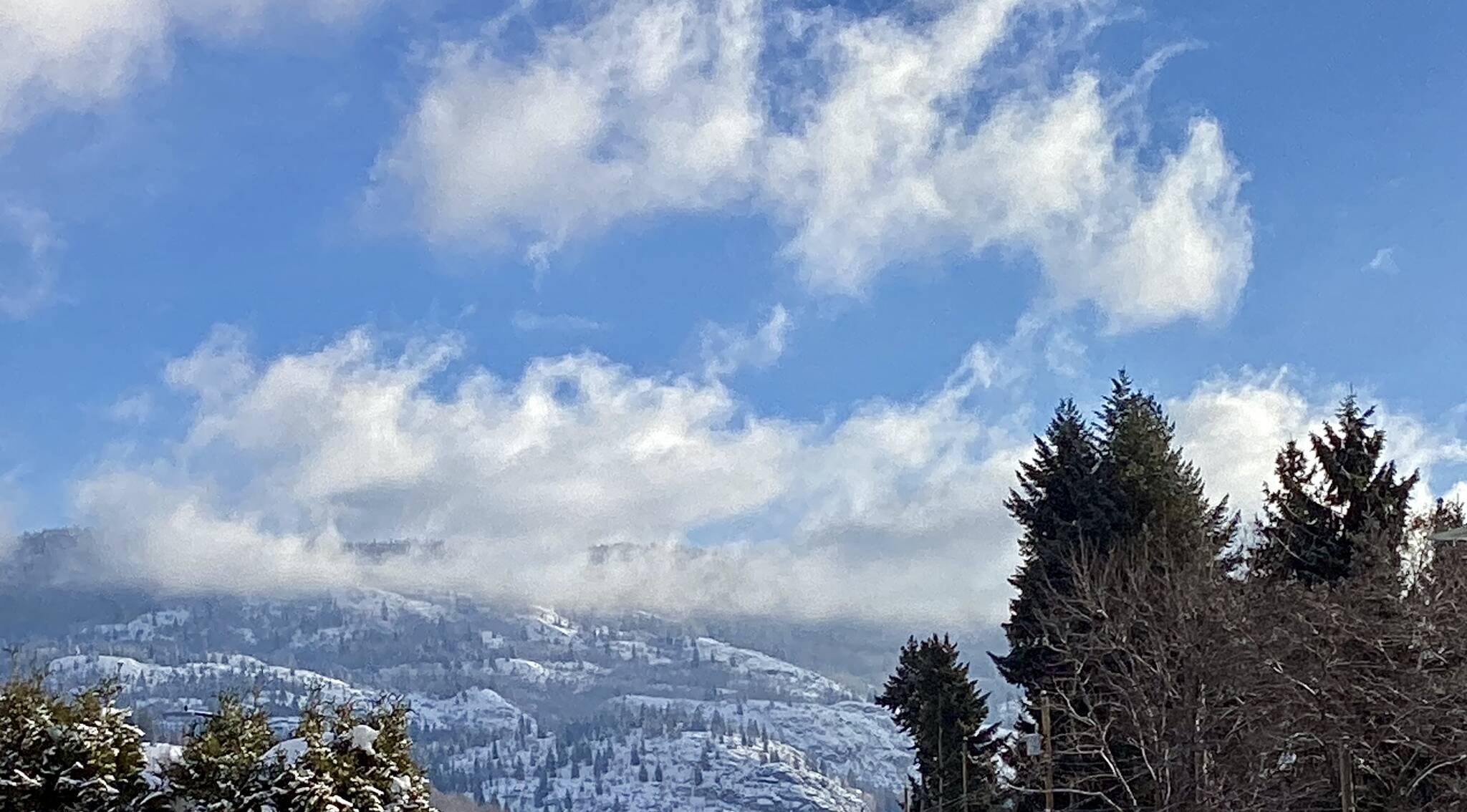The photograph captures a serene landscape dominated by a vast blue sky interspersed with floating, thin, puffy clouds. In the lower right corner, a cluster of tall, dark green pine trees stands, some appearing bare with twigs protruding. Contrastingly, the lower left corner features pine trees adorned with snow-covered branches, adding a touch of winter's charm. The scene extends into the distance where low, rolling hills spread out, dotted with scattered, narrow pine trees typical of far northern tundras. These snow-covered hills, marked by crevices, add a subtle texture to the background. The overall composition creates a harmonious blend of snowy and green elements against the backdrop of a crisp, clear sky, offering a picturesque glimpse into a tranquil, mountainous terrain.